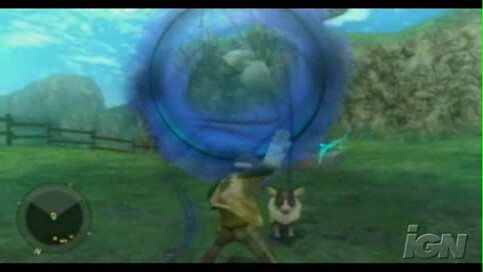This image is a low-quality, blurry screenshot from a video game, bearing a watermark of IGN in the bottom right corner. The scene depicts a character standing in the center, facing away from the camera with legs spread and arms extended, wearing a brown coat with blue sleeves and green pants, appearing to cast a glowing blue, circular energy field above him. To the right of the character is a goat, facing the camera, with a brown head, white nose, white ears, and a white body. The setting includes green grass in the foreground, a wooden fence on the left side, and a backdrop of trees, mountains, and blue skies with scattered clouds. In the lower left corner, there is a plain, dark-gray compass or radar-like circle with an indistinguishable highlighted section, possibly indicating direction. The overall aesthetic hints at a game involving creature capturing and training, reminiscent of Pokémon but distinctively different.